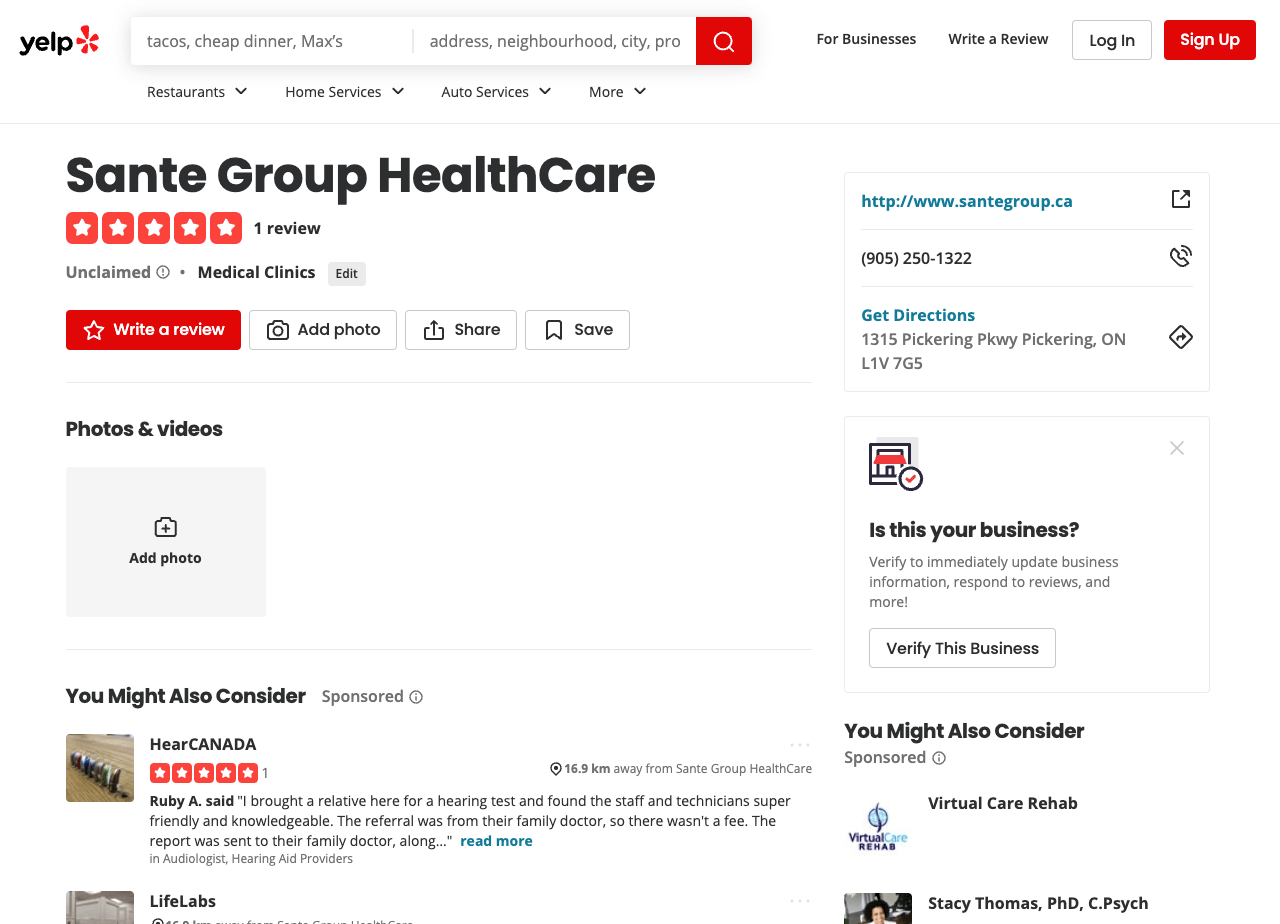This image is a detailed screenshot of a Yelp listing for a healthcare company called Sante Group Healthcare. At the top, the image features the Yelp logo alongside a search bar and various links including options for businesses, writing a review, logging in, and signing up. Directly below, there is a menu bar offering categories such as restaurants, home services, auto services, and more.

The central portion of the screenshot prominently displays the business name, Sante Group Healthcare. The company is highly rated, holding a five-star rating based on one review, but the business remains unclaimed and is categorized under medical clinics. Directly beneath this information, there are four interactive buttons allowing users to write a review, add photos, share, or save the listing.

Further down, there is a section titled "Photos and Videos" which includes an option to add photos, though currently, there are no pictures available. At the bottom of the main section, there is a "You Might Also Consider" section, identified as a sponsored area, featuring recommendations for other businesses—HERE Canada and Life Labs.

On the right pane of the screenshot, essential business details such as the company website, phone number, address, and a link for directions are displayed. There is also a box prompting the business owner to verify the listing with the message, "Is this your business? Verify this business." Below this prompt, another sponsored "You Might Also Consider" section appears, suggesting Virtual Care Rehab and Stacey Thomas, PhD C-Psych as alternative options.